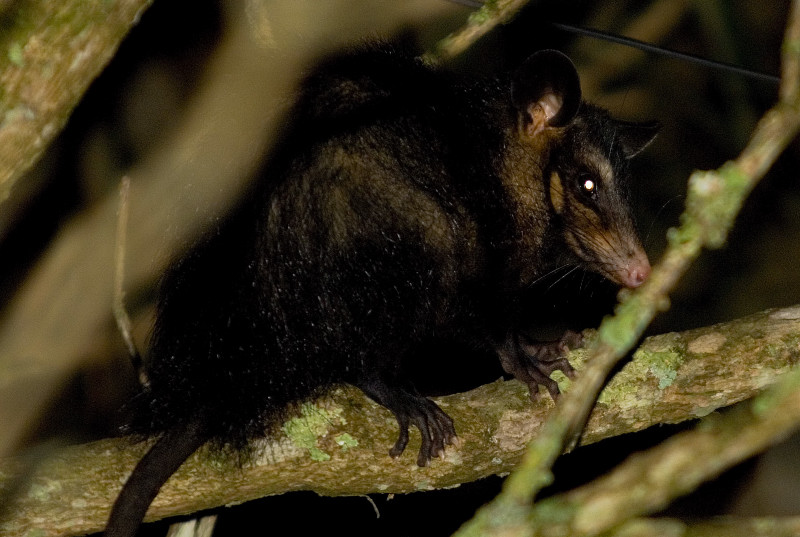The photograph captures a small mammal, likely a possum, perched or moving along a branch in what appears to be a nighttime setting, suggested by the use of flash and the notable eye reflection, resulting in a white circle. The animal's defining features include dark, almost black, fur, a pink nose, and pointed ears similar to those of a cat. Both of its rear feet, equipped with small claws, are clinging to the branch, alongside its long, rat-like tail. The branches in the image are brown with patches of green moss and there are several others visible, though slightly blurred and out of focus due to the nighttime conditions. The background remains largely indistinct, enhancing the sense of the animal creeping stealthily through the nocturnal scene.